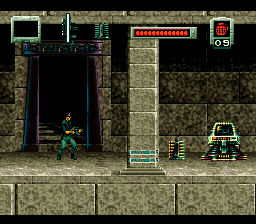In this vintage side-scrolling shooter video game image, a character dressed in a blue military outfit is seen moving from left to right across a cement-like environment. The character is armed with a gun, emphasizing its action-packed nature. To the right of the character, there is a computer, hinting at an interactive or technological element within the game. Above, a horizontal health bar filled predominantly with red is visible, with only a small portion depleted at the top, indicating the character's current health status. Besides the health bar, there is a red grenade icon marked with the number nine, likely representing the number of grenades available. Other various symbols and indicators line the top of the screen, providing additional game information. The character appears to be emerging from a doorway and descending a staircase, poised for the next segment of the level. The overall graphical style reflects the game's older origins, lacking the detailed realism of contemporary video games, yet retaining a distinct nostalgic charm.